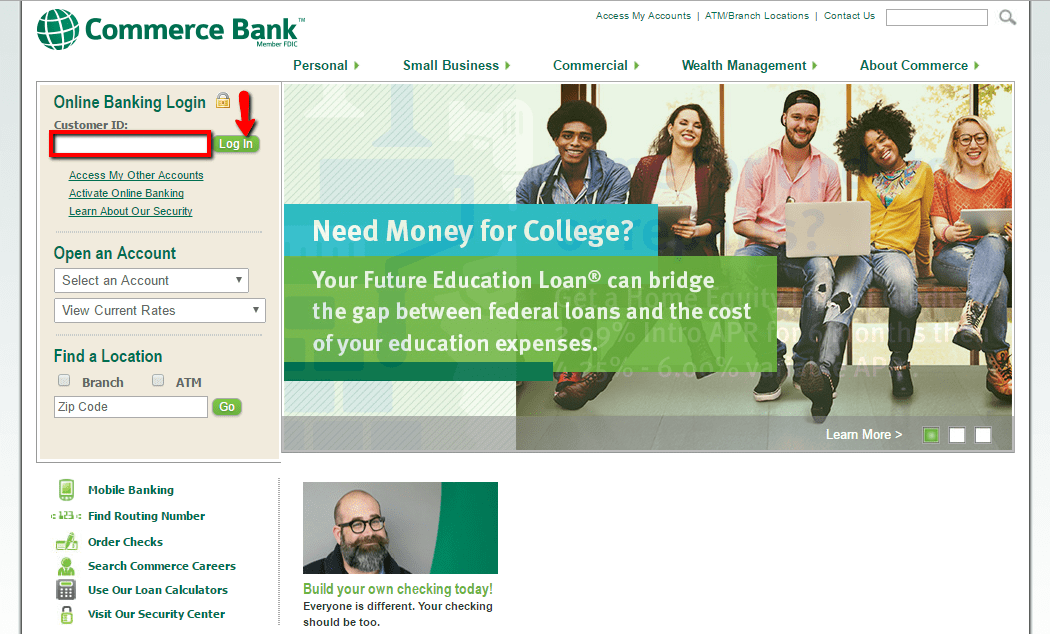The image is a screenshot from a website for Commerce Bank. At the top of the webpage, "Commerce Bank" is prominently displayed in green text alongside a green globe featuring a white checkerboard pattern.

Below this header, there are numerous drop-down menus labeled "Personal," "Small Business," "Commercial," "Wealth Management," and "About Commerce." These menus provide various options for navigating the bank's services.

The central section of the webpage features a picture of five people sitting on a bench, all smiling. Three of the individuals have an open laptop on their laps. Above them, a teal rectangle contains the heading "Need Money for College?" Underneath, within a green rectangle, it states, "Your future education loan can bridge the gap between federal loans and the cost of your education expenses."

Further down the page, there's an image of a mostly bald man wearing black circular glasses, with a beard and mustache. Adjacent to his photo is a call-to-action text saying, "Build your own checking today."